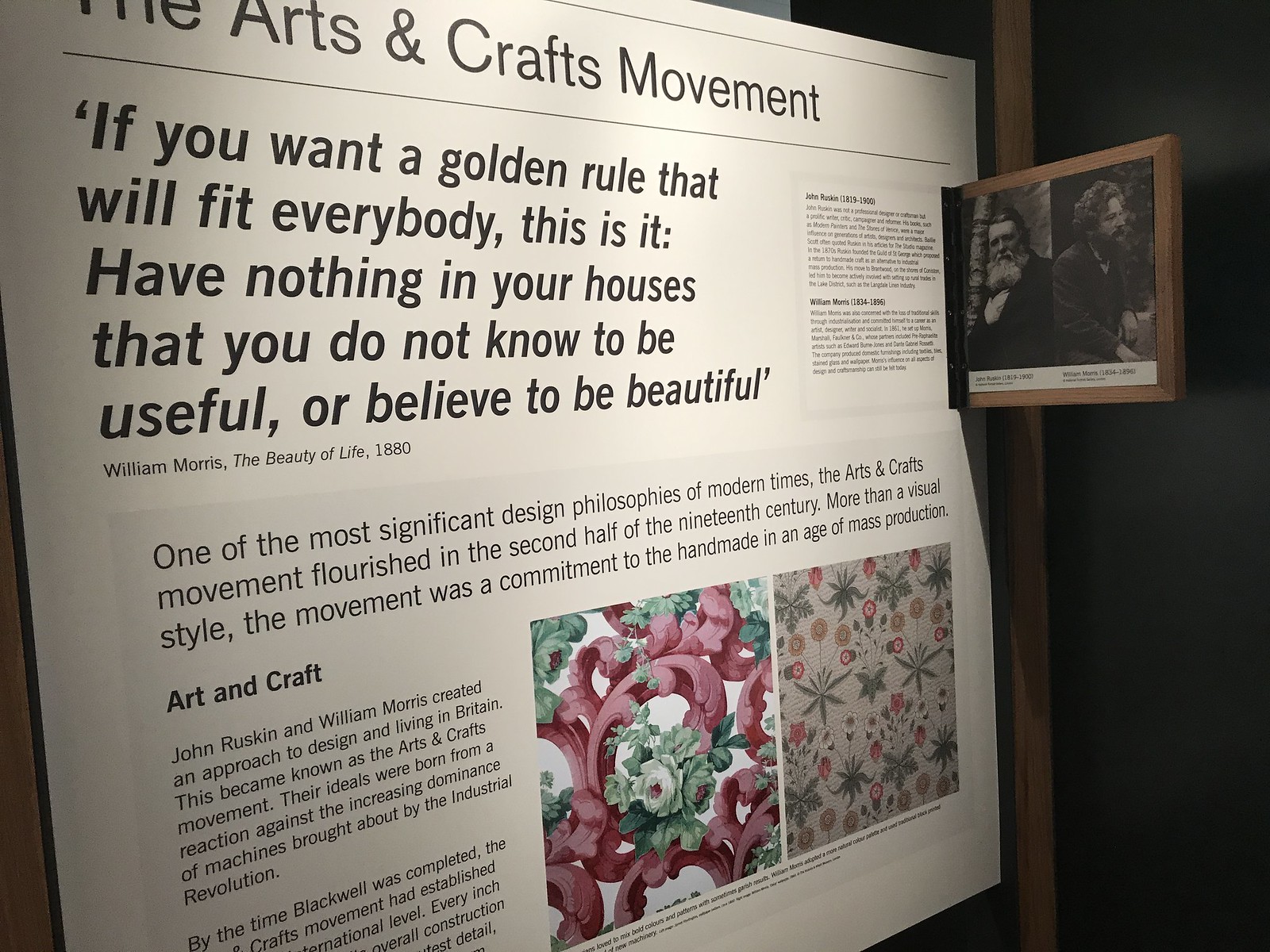This image captures a museum exhibition poster detailing the influential Arts and Crafts Movement. At the top of the poster, a significant quote by William Morris from "The Beauty of Life," 1880, reads: "If you want a golden rule that will fit everybody, this is it. Have nothing in your houses that you do not know to be useful or believe to be beautiful." Below this, the text elaborates on the movement, describing it as "one of the most significant design philosophies of modern times." It explains that the Arts and Crafts Movement, which flourished in the latter half of the 19th century, was dominated by a commitment to handmade craftsmanship in response to the mechanical production brought by the Industrial Revolution. Founders, John Ruskin and William Morris, envisioned a design approach that balanced utility and beauty, leading to an enduring international influence. 

The bottom part of the poster is obscured, but the left section includes a brief mentioning Blackwell's completion, reflecting the Movement's established international presence. The right side features two floral pattern images exemplifying the Arts and Crafts style: one with a detailed three-dimensional floral design and another with a simpler, gift wrapping-like pattern of red bubbles and green star shapes against a beige background. Adjacent to these visuals is a framed photograph showing two men, believed to be John Ruskin and William Morris, though the captions are too small to confirm. This exhibition is likely part of a larger museum display dedicated to exploring the legacy of the Arts and Crafts Movement.